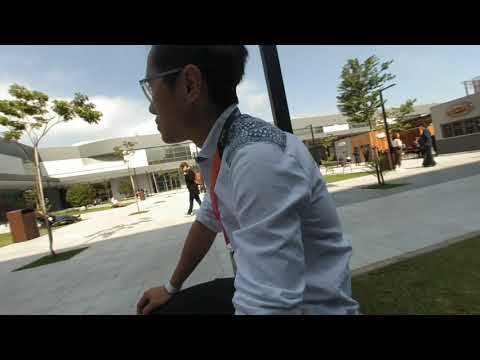In this photograph, there is a man with glasses, wearing a long-sleeved white collared shirt with sleeves rolled up to his elbows. He has an orange lanyard around his neck and a white wristband on his left arm. The man appears to be Asian and is seen looking to his left. He is seated outdoors, possibly on a college campus during a break between classes. His right hand rests on his knee. The background reveals a modern architectural setting, featuring white pavement, trees, and a mix of people walking and standing around, some with backpacks suggesting a student population. The surroundings include buildings that are mostly white and appear to be two stories high with glass entrances. The blue sky with scattered clouds adds to the ambiance of the scene. Additionally, there is a brown garbage can visible nearby, reinforcing the campus-like environment.